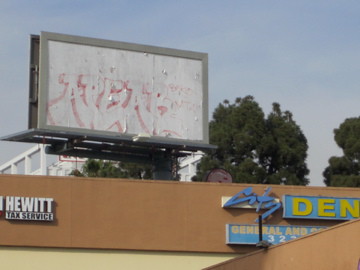The image features a weathered billboard, predominantly white with remnants of red text or imagery, suggesting the original message has been partially torn off. The billboard, possibly a traditional one rather than electronic, stands amidst several green trees with a hazy, bluish sky overhead that evokes a nostalgic, vintage feel. In the foreground, a brown wall extends horizontally, adorned with white graffiti spelling "Hewitt," likely referring to a tax company. Additionally, a blue sign with yellow lettering displaying "DEN" is visible. The photo appears slightly blurred, possibly captured from a moving vehicle, contributing to the overall lack of fine detail.